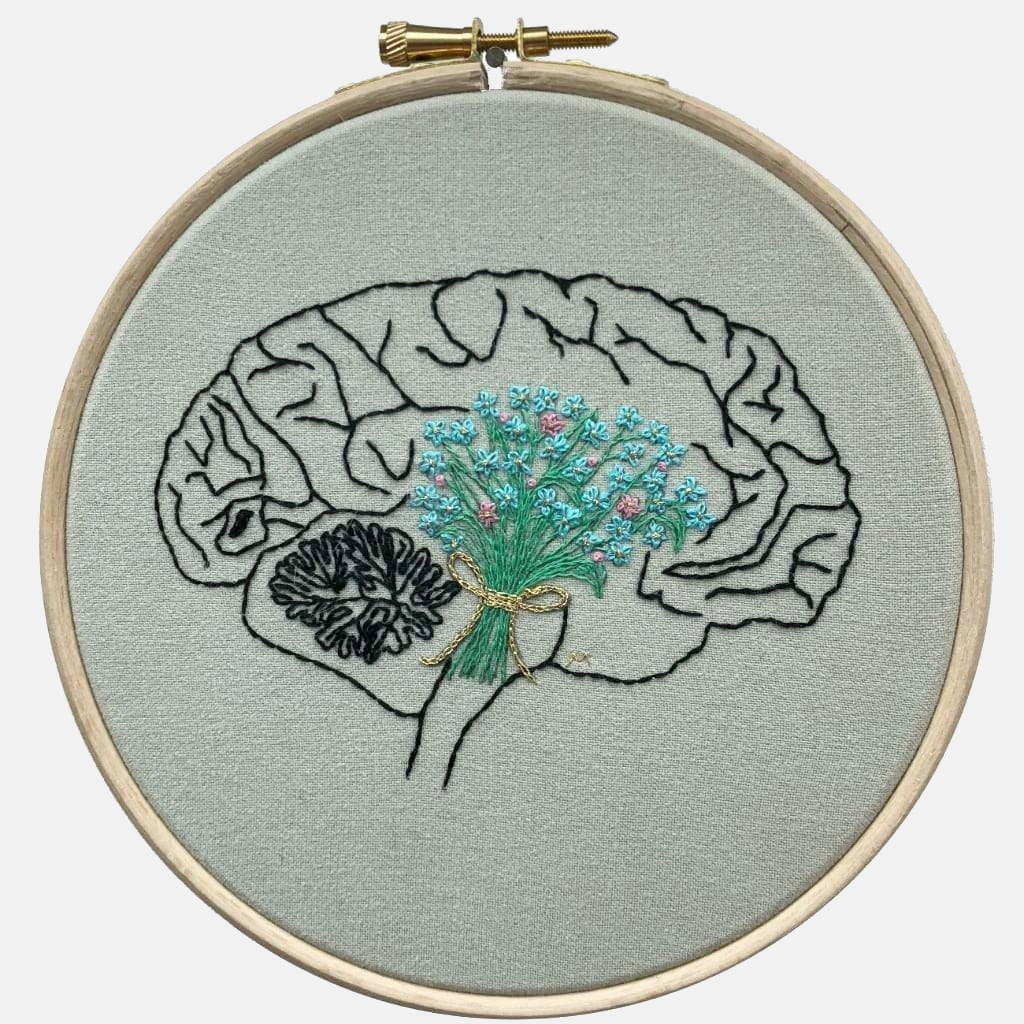The photograph showcases a hand-embroidered piece of fabric secured in a light brown wooden embroidery hoop, characterized by a pair of bronze clasps fastened with a bronze screw and bolt at the top. The image is square-shaped with equal dimensions on all sides and set against a light gray background. The fabric within the hoop is a light gray heather material, providing a subtle contrast to the intricate black thread embroidery that outlines the form of a human brain at the center. Adding a touch of color and vibrancy, a small bouquet of green and blue flowers is delicately stitched atop the brain, showcasing the craftsmanship and attention to detail in this unique and creative piece. Though reminiscent of stained glass in its design, the artwork is entirely crafted from thread, melding traditional embroidery techniques with imaginative and modern motifs.